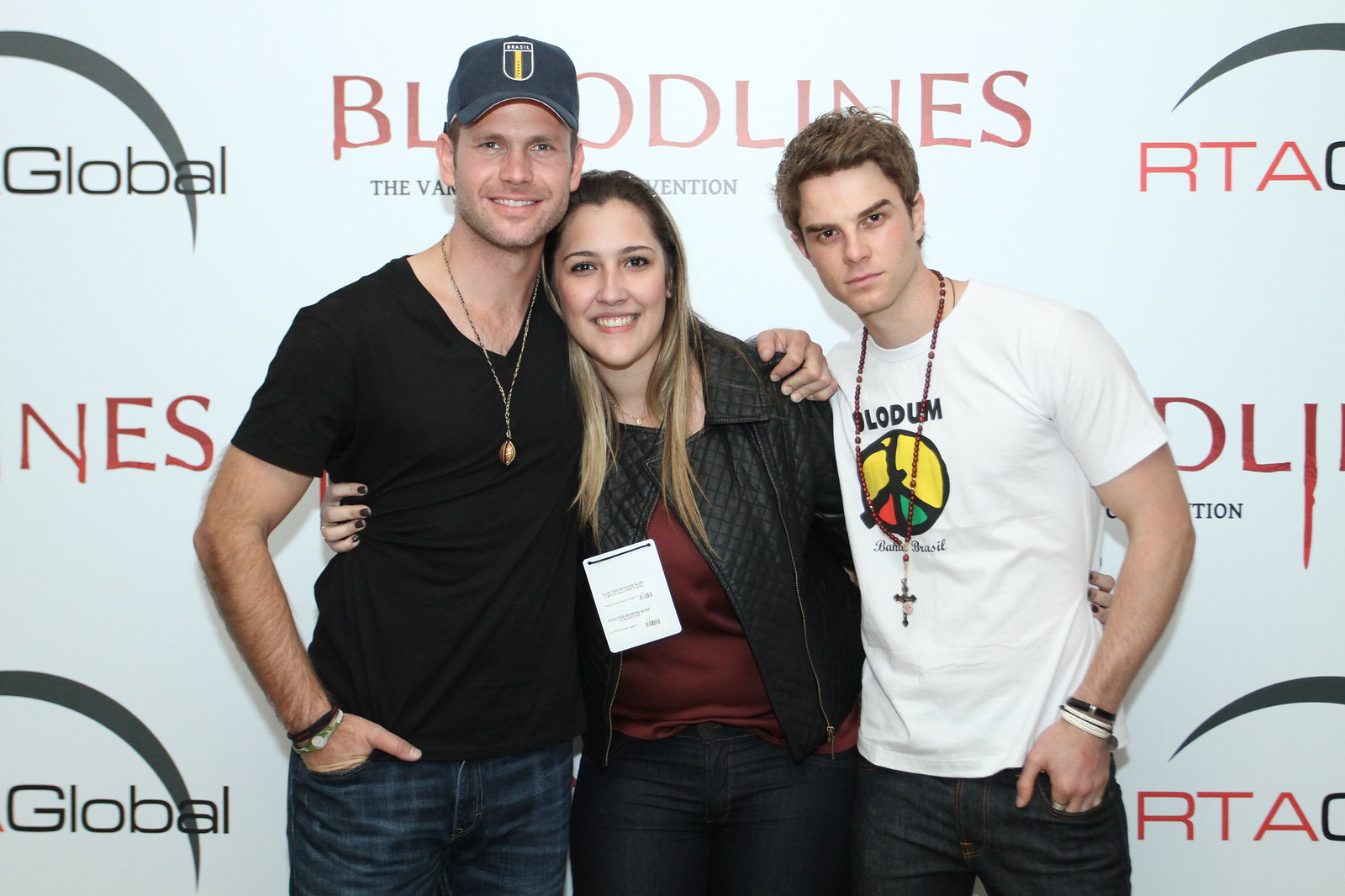The vibrant and clear image captures three young people posing closely in front of a white banner that reads "Global Bloodlines" in red and black writing. On the left stands a cheerful young man with a black V-neck shirt, blue jeans, a black hat, and bracelets adorning his wrist, while his hands rest casually in his pockets. The woman in the middle, with her dirty blonde hair cascading down, sports a black jacket over a burgundy shirt, along with dark jeans. She has her arms wrapped affectionately around both men. To her right is another young man, wearing a white shirt emblazoned with "Bloodham" and a peace sign in yellow, green, and red, along with dark jeans. He accessorizes with a long necklace featuring a cross and bracelets on his wrist. The trio appears to be enjoying each other's company at what seems to be an event, as they radiate warmth and camaraderie.